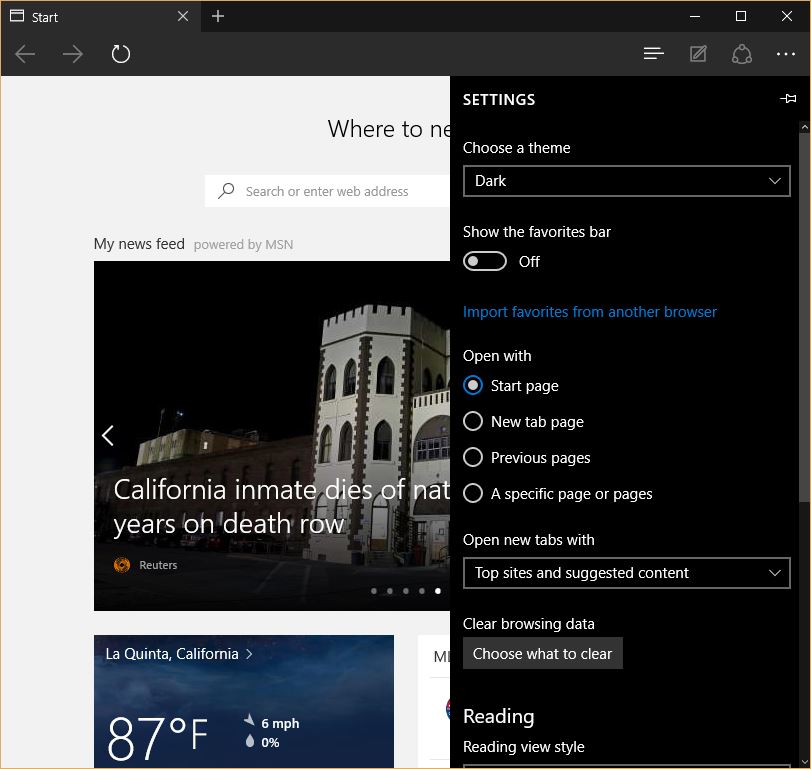This vertical image, sourced from a webpage accessible via computer, provides a detailed view of a standard web browser interface. At the very top, a gray, short rectangular bar includes the "Start" button on the upper left-hand side, accompanied by an icon. An "X" follows this, shifting to a thinner block line extending across the screen, ending with a plus sign. On the upper right-hand corner are the minimize, maximize, and close buttons.

Beneath the "Start" section, the gray color resumes, showcasing left and right navigation arrows, a refresh button, and additional icons to the right. The backdrop features a light gray hue where only fragments of elements are visible, including part of a phrase that reads "where to" and partially obscured letters "N" and "E."

A prominent white search bar is displayed, accompanied by a section labeled "My News Feed powered by MSN." Within this news feed, a headline reads "California inmate dies of [incomplete]," suggesting a breaking news story. Another segment shows the current weather in La Quinta, California.

Additionally, a black, horizontally oriented rectangle has popped up in the middle of the screen, indicating an active settings menu. This menu allows the user to choose a theme (e.g., dark mode), show the favorites bar, import favorites from another browser, and set the browser's start page preferences, such as opening with the start page, a new tab page, the previous page, or a specific page. It also includes options for opening new tabs with top sites and suggested content. Lastly, the menu provides settings for clearing browsing data and selecting specific elements to clear, alongside reading preferences.

The image overall offers a comprehensive glimpse into a user's interaction with their web browser settings and interface.